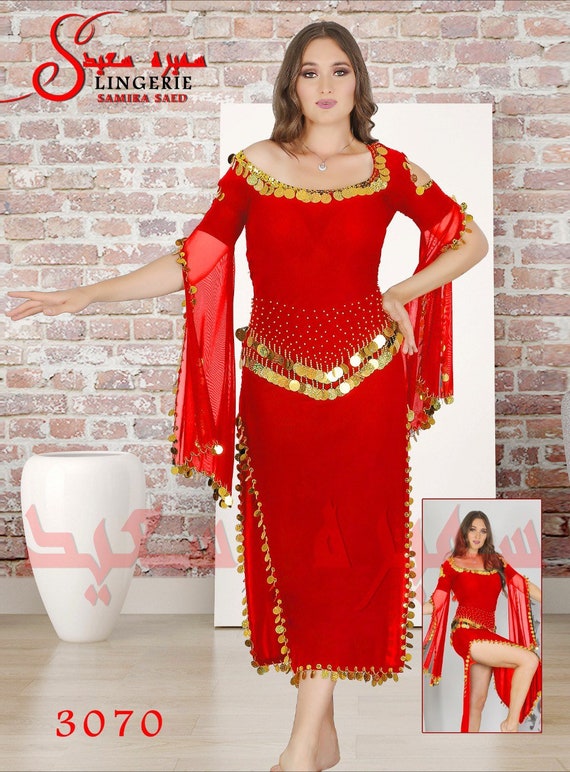This poster features a woman, Miss Samira Syed, modeling a Middle Eastern-inspired, red see-through gown adorned with golden accents around the collar, sleeves, waist, and sides. The gown extends just above her ankles. Above her stands the brand name in bold black lettering with "lingerie" and "Samira Syed" prominently displayed in red. Miss Syed is posed against a white cutout board that's propped against an aged brick wall on a wooden floor. To the left, a white vase approximately two to three feet tall adds a decorative element. There is Arabic text in transparent red font at the bottom. Additionally, a smaller inset features Miss Syed in the same dress, lifting one leg. The numbers "30, 70" are seen in the lower left corner of the poster.